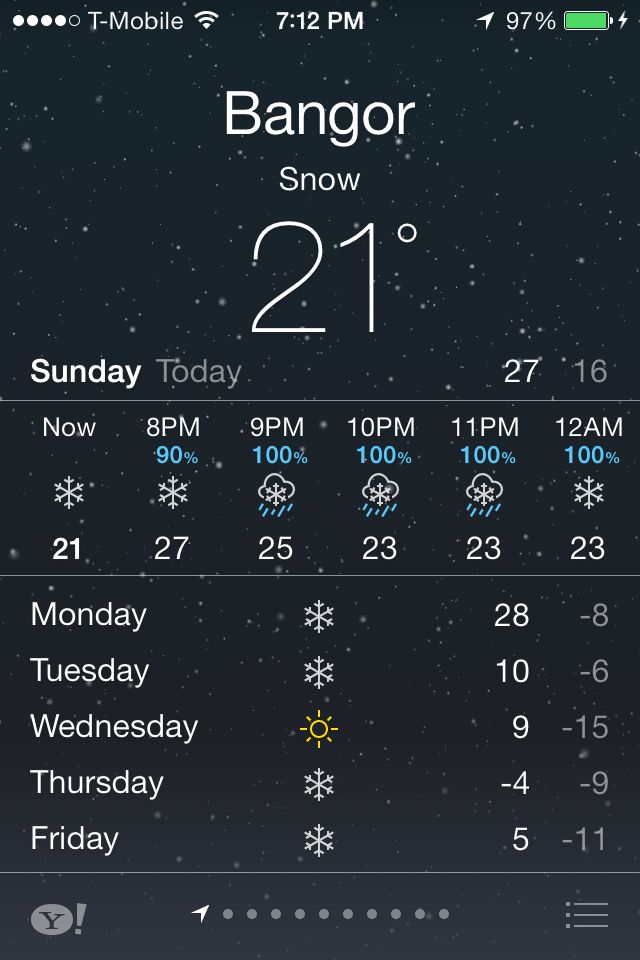The screenshot showcases the Yahoo Weather app running on a smartphone. The top section of the screen displays various phone status indicators, including a T-Mobile carrier label, a Wi-Fi signal icon, a time display showing 7:12 p.m., and a battery life indicator at 97%. The app interface focuses on weather details for Bangor, where the background depicts a dark, snowy sky. The current temperature is prominently shown as 21°F, with a notice indicating snow.

A highlighted section identifies Sunday as the selected day, in contrast to other days that are grayed out. The temperature for Sunday is shown to be 27°F. Further down, a detailed hourly forecast is visible, spanning from 8 p.m. to 12 a.m., indicating a high snow probability of 90% at 8 p.m., with the percentages for subsequent hours not fully visible.